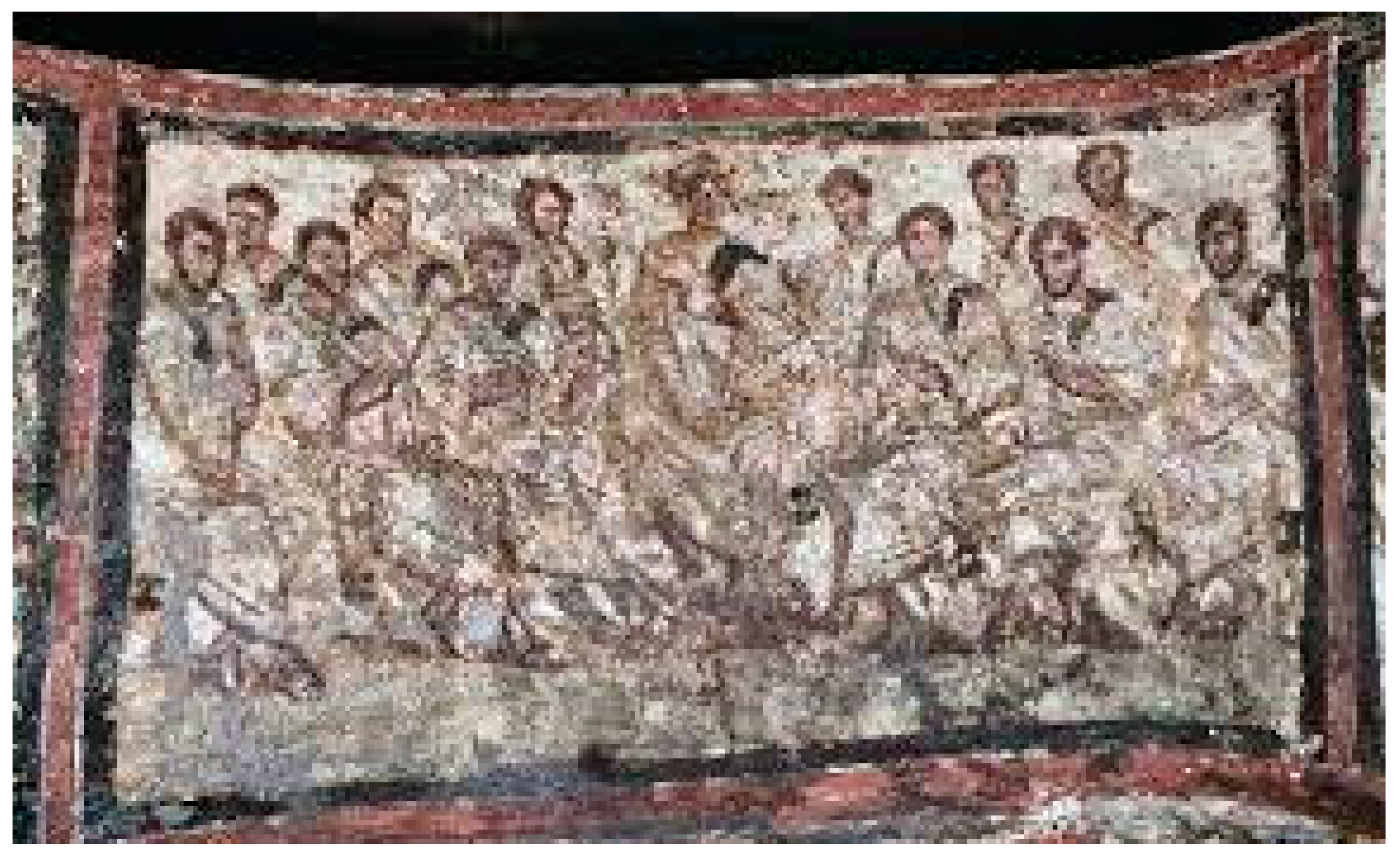The image depicts a highly pixelated, ancient mosaic or mural on a curved wall, displaying a group of men adorned in white robes or togas. These figures, possibly from Roman times, share short-cropped hair and seem to be arranged in a manner suggesting a focal point at the center. The mosaic appears to be framed with a black border enveloped by a red one, and is part of a sequence of interconnected scenes, reminiscent of an ancient comic strip. The photograph captures only part of the mural, hinting at additional scenes extending beyond the image. The artwork seems weathered and dingy, possibly indicating age or exposure to elements.